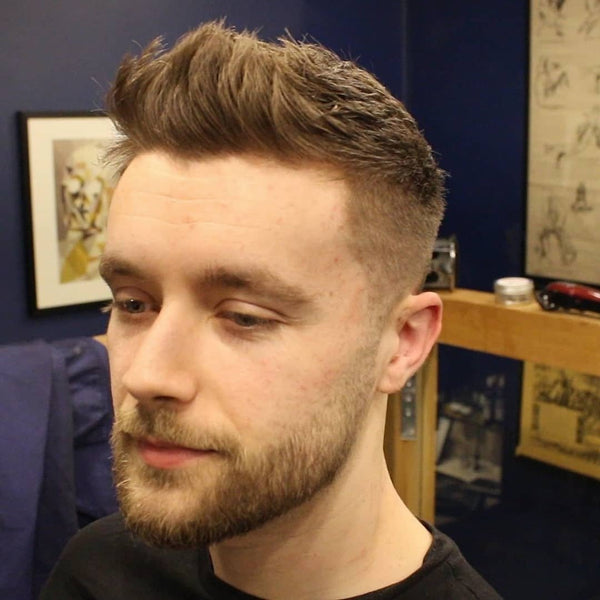The photo is a close-up of a young white man, around 24 to 25 years old, with a neutral expression, gazing off to the bottom left. He has blue eyes, long thin blonde eyelashes, slight wrinkles under his eyes, and light brown hair styled with gel, slicked back and upwards. His beard and thin mustache are also light brown. He's wearing a black T-shirt, and only his head and neck are visible. There is a royal blue wall in the background, adorned with two portraits: one on the left featuring a skull and a longer one on the right with several illustrations. Below the right portrait, there's a thin wooden surface with objects on it, and above his left ear, there's a small silver radio. The setting appears like a barber shop or a place where people showcase their haircuts.